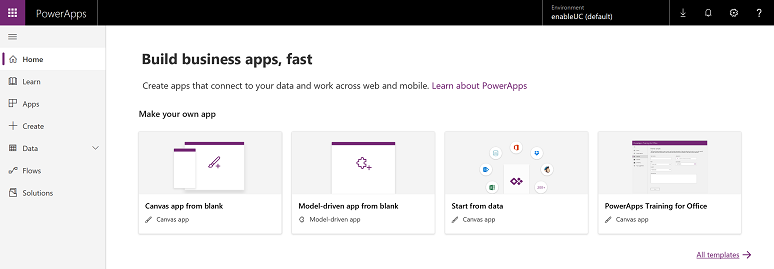The image is a screenshot from a webpage related to Power Apps, showcasing the application's interface and key features. The top section of the webpage is dominated by a black rectangular banner containing the Power Apps logo—a purple square with nine smaller squares arranged in the shape of a cube—and the text "Power Apps." 

Below the banner, there are several icons including a download button, a bell, a gear, and a question mark. Just below this row of icons, the text "Enable UC (Default)" is visible. 

Centrally, in bold letters, the webpage proclaims "Build Business Apps Fast," followed by a subheading, "Create apps that connect to your data and work across web and mobile. Learn about Power Apps." The phrase "Learn about Power Apps" is in purple, indicating it is a clickable link.

Further down, the webpage invites users to "Make Your Own App" and provides four actionable options in separate boxes. These options are:

1. "Canvas App from blank" with a subtext "Canvas App."
2. "Model-Driven App from blank" with a subtext "Model Driven App."
3. "Start from Data" with a subtext "Canvas App."
4. "Power Apps Training for Office" with a subtext "Canvas App."

Each of these boxes appears to offer guided steps or templates for creating different types of apps within the Power Apps platform.